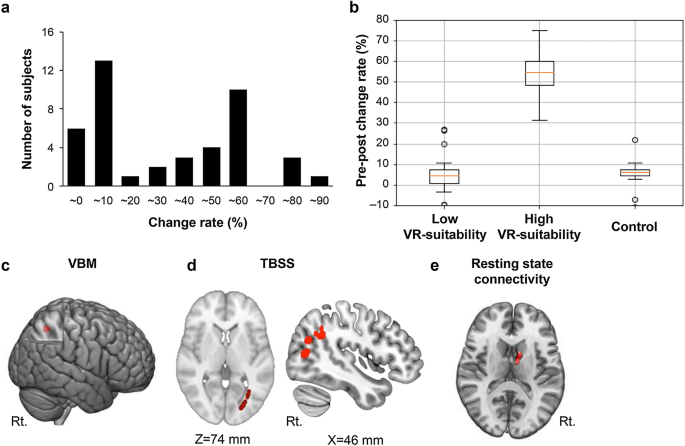The image showcases the results of a medical study displayed against a clean, white background with no official border. In the upper left corner, labeled A, is a bar graph depicting the number of subjects versus the change rate percentage, illustrated with numerous black bars. To the upper right, labeled B, is a line graph that presents pre- and post-change rate percentages across categories such as low suitability, high suitability, and control, with the y-axis ranging from -10 to 80. Along the bottom are three detailed black and white scans of the human brain, labeled C, D, and E. These scans indicate different views: C shows the VBM (right view), D shows the TBSS (top view), and E shows the resting state connectivity (scanned view), with specific features highlighted by red dots.